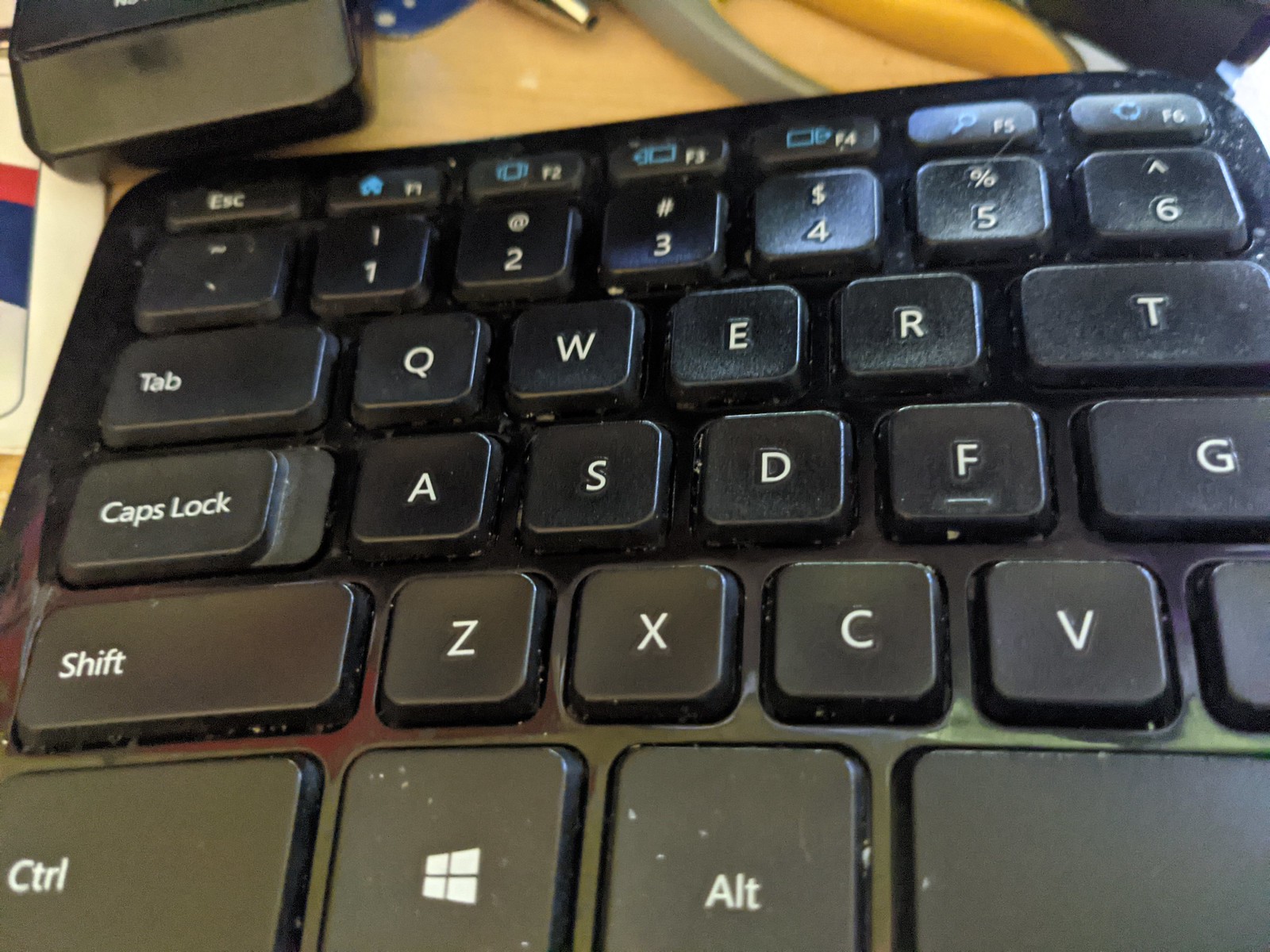The image is a detailed close-up of the upper left quadrant of a black computer keyboard, prominently displaying keys with white text. It spans from the Escape key on the outer left through the F6 key, covering keys like Tab, Caps Lock, Shift, Control, and parts of the number row (1 through 6) as well as the letter rows (Q to T, A to G, and Z to V). Notably, part of the key adjacent to the G is partially visible but not fully shown. The surrounding area also reveals other elements: a segment of a black wire and a pen resting on a light-grained wooden surface, hinting at a desk setup. Additionally, there's an object resembling a white envelope with blue and red stripes in the background, further enriching the scene.